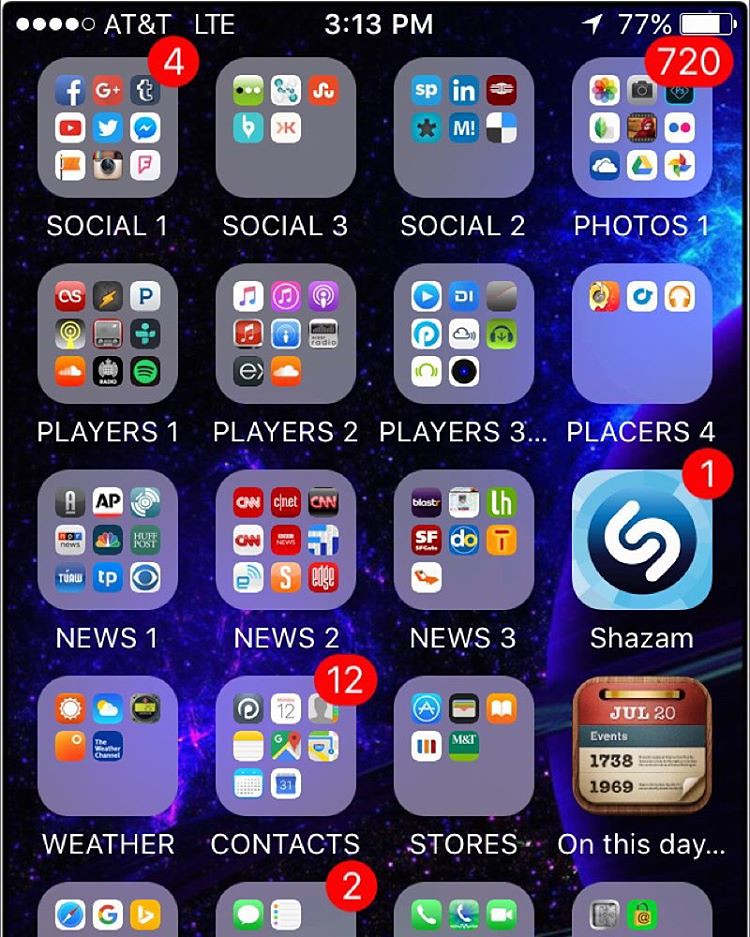A detailed screenshot of an iPhone home screen showing a well-organized layout with most apps grouped into folders. In the upper-left corner, the status bar displays the carrier "AT&T," accompanied by "LTE," indicating a fourth-generation cellular network, with the signal strength showing four out of five solid white circles, and the rightmost circle outlined in white. The current time is 3:13 PM. To the upper right, the location services icon, a white arrow, is visible, along with the battery level at 77%, represented both numerically and graphically with a bar inside a white battery icon.

The apps on the home screen are primarily organized into several distinct groupings, each labeled appropriately. Notable apps outside these groups include Shazam and an app titled "On This Day," which is truncated with an ellipsis. Clearly labeled folders encompass various categories: "Social," "Photos," "Players," "Places," "News," "Weather," "Contacts," and "Stores." The layout displays four full rows of app icons and folders, with a fifth row partially visible at the bottom of the screen.